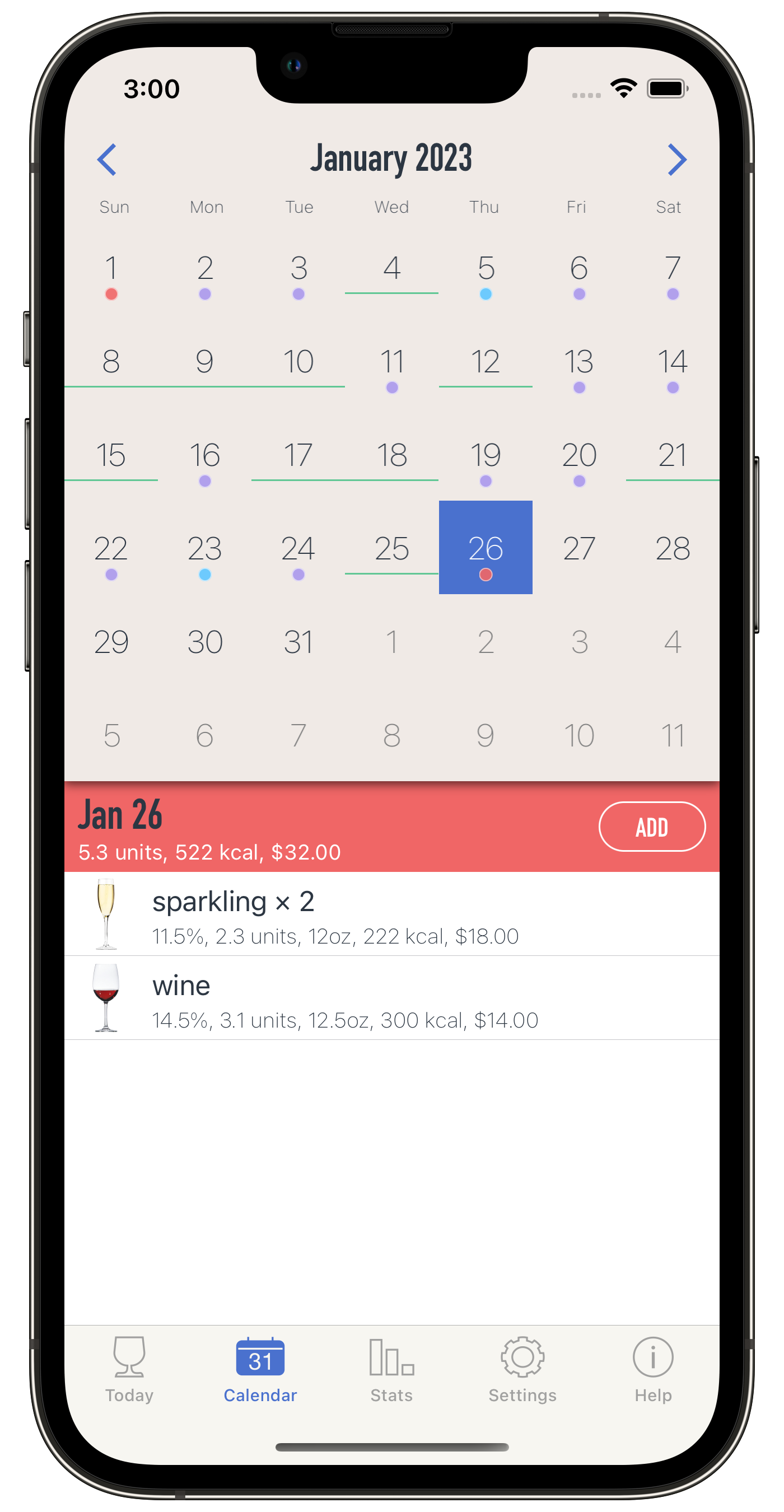The image depicts a smartphone with a black casing, resembling an iPhone. The screen is facing forward, featuring the dynamic island at the top. The surrounding buttons are visible along the phone's edges. The background of the image is white.

At the top-left corner of the screen, the time is displayed as 3:00. On the right side, there are four small gray dots in a row, followed by the Wi-Fi signal indicator, and the battery icon. Below this top section, there are two blue arrows pointing left and right, each positioned on their respective sides.

Centrally, in bold black text, the date "January 2023" is displayed with a capital "J". Below this, the calendar layout for January is shown, starting with January 1st marked as a Sunday. This date has a small red dot underneath it.

Subsequent dates contain various markers:
- January 2nd and 3rd have purple dots.
- January 4th has a green line.
- January 5th has a turquoise dot.
- January 6th and 7th have purple dots.
- January 8th, 9th, and 10th have a green line.
- January 11th has a purple dot.
- January 12th has a green line.
- January 13th and 14th have purple dots.
- January 15th has a green line.
- January 16th has a purple dot.
- January 17th and 18th have green underlines.
- January 19th and 20th have purple dots.
- January 21st has a green line.
- January 22nd has a purple dot.
- January 23rd has a turquoise dot.
- January 24th has a purple dot.
- January 25th has a green line.
- January 26th is uniquely marked with a blue square background, containing the date "26" in white text with a red dot underneath.

The text "January 26: 5.3 units, 522 Kcal, $32 add" is present, indicating specific details related to that date. Additionally, there's a note: "sparkling times two," referring to wine.